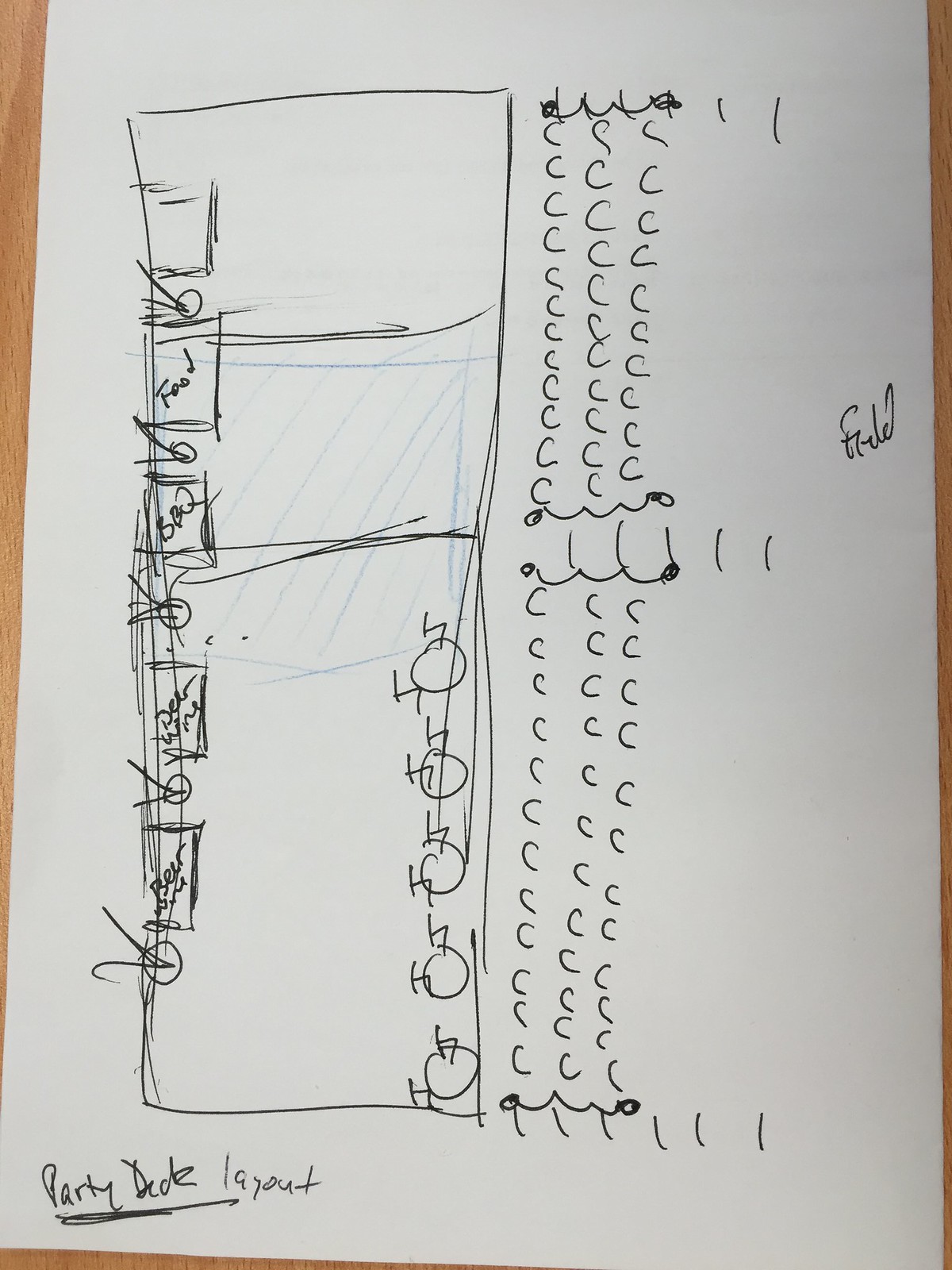This image captures a meticulous, handwritten layout on a white piece of paper, detailing the setup plan for what appears to be a party. The lower-left corner of the paper features the handwritten title "Party Decor Layout," which is underlined for emphasis. 

In the main section of the paper, there's a large rectangle sketched out, likely representing the party room. Within this room, several rectangular tables are drawn. The first table at the very top is unmarked, while the second is labeled "Food." The third table is marked "BBQ," and the labels on the following two tables are difficult to decipher.

Between these rectangular tables, there is a drawing of a plant, rendered simply in pen, suggesting a decorative element. 

On the right side of the room, there are five round tables, each accompanied by approximately two chairs. 

On the entire right edge of the page, the person has drawn three vertical rows of the letter 'C,' followed by another three rows below. These rows have squiggly marks adjacent to them, possibly indicating a counting mechanism. 

Additionally, a word appears on the far right side of the page that seems to say "free."